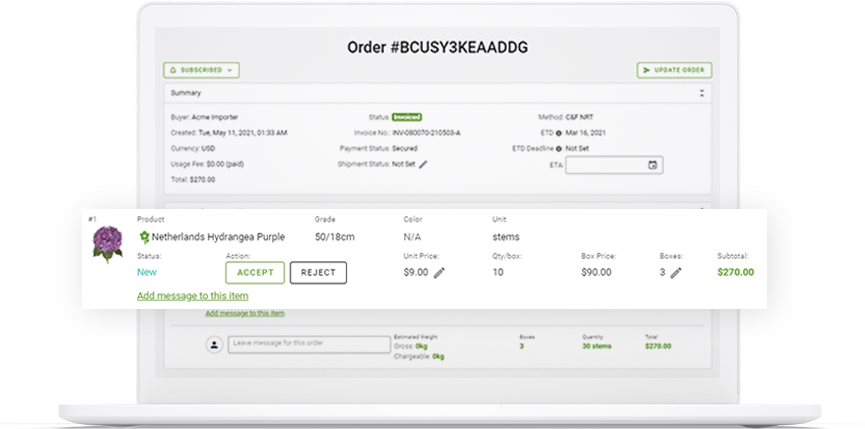This horizontal image appears as a screenshot taken from a computer or smartphone application, likely against a white background. The image showcases a digital interface framed by multiple layers of gray borders. At the top, within one of the darker gray borders, the order number "BCUSY3KEAADDG" is displayed in black text.

To the left, there's a green button labeled "Subscribed," and to the right, a green button with a small triangle labeled "Update Order." Below these buttons, the order summary is detailed, providing comprehensive information about currency, usage fee, total cost, order status, invoice number, payment status, shipment status, shipping method, and estimated time of arrival (ETA). An icon of a calendar is also visible to indicate the ETA.

Prominently displayed in a large, white, rectangular pop-up box is specific product information. The product listed is "Netherlands Hydrangea Purple," accompanied by its status and available actions such as "Accept" or "Reject." The subtotal for this product is $270, clearly marked within the interface.